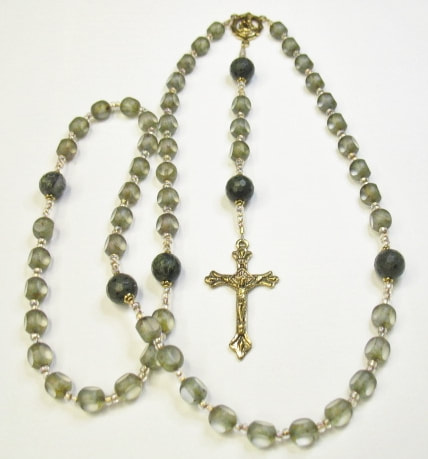This image captures a serene and evocative photograph of rosary beads meticulously arranged on an off-white surface. The rosary features an elegant gold crucifix centrally displayed, highlighting its significance and old-world charm. The beads predominantly showcase a jade green hue, interspersed with six distinct dark blue beads. These beads create a striking contrast, enhancing the visual appeal. The rosary's arrangement forms a complex pattern, with the strands overlapping and creating two distinct circles—one smaller on the left and a larger one on the right. The meticulous positioning of the beads and the crucifix imbues the photo with a sense of peaceful contemplation and timeless beauty.